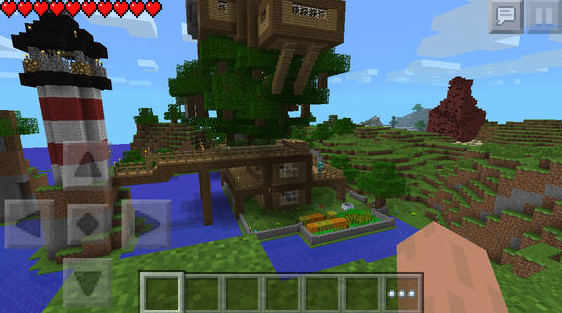The image depicts a detailed Minecraft village scene in a mobile version of the game. At the bottom of the screen, there is an inventory bar displaying seven squares numbered 1 through 7. On the left side of the screen, navigation arrows for left, right, up, and down, along with a central button, can be observed. The top left corner shows a health bar with ten hearts.

Prominently featured on the left side of the image is a meticulously crafted lighthouse, constructed with alternating layers of white and red blocks. The lighthouse is supported by a stone fence and crowned with a brown top. Adjacent to the lighthouse, there is a wooden bridge that leads into a window, providing access to the inside structures.

Surrounding the village, lush green grass and diverse terrain can be seen, including grassy hills that transition into dirt and a towering mountain in the background. The sky is a vivid blue filled with fluffy white clouds, and a serene blue river meanders through the landscape. Nested among the natural scenery is a wooden treehouse, seamlessly blending into the idyllic setting.